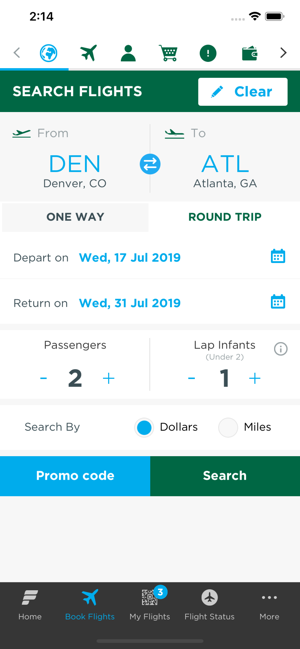The top section of the image features a navigation bar with six distinct icons arranged horizontally: a globe, an airplane, a user profile, a shopping cart, a notifications bell, and a wallet. On the far left of this bar is a back arrow, while a white forward arrow appears on the far right. 

Beneath this bar lies a green search bar labeled "Search Flights," complemented by a white "Clear" button situated to the right, and a pencil icon positioned to the left of the search bar. 

Immediately below this green bar is a grey input area labeled "From" on the left and "To" on the right, which indicates the departure and destination fields. The specific departure location listed is Denver, Denver, Colorado, accompanied by an associated icon. 

[The rest of the image description was cut off. The image may include additional details such as further fields for trip type or more specific travel information.]